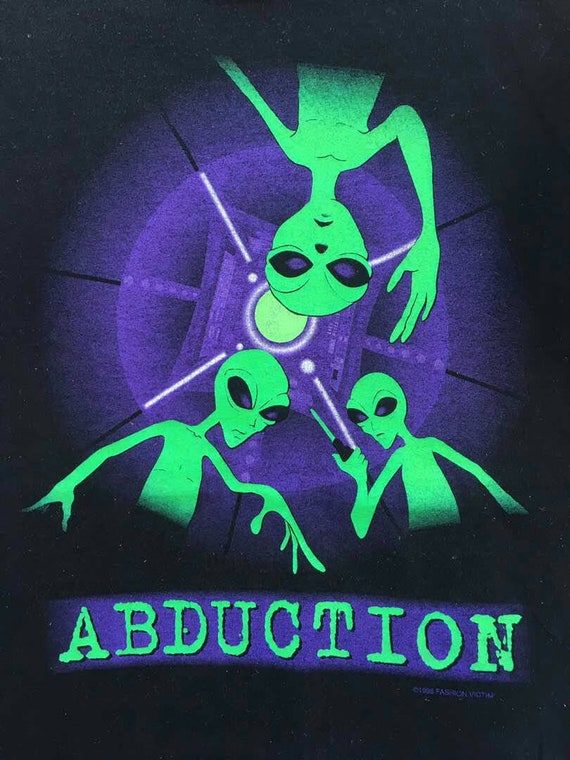This detailed animated image portrays three green aliens set against a predominantly black background, reminiscent of a poster. The backdrop, a contrasting rectangular frame, highlights a vivid purple circular area at its center, where the aliens are prominently featured. Notably, one alien emerges upside down from the top, its bulbous light bulb-shaped head with disproportionately large black eyes positioned centrally. The other two aliens stand upright, flanking the lower left and right corners of the image. The right-side alien brandishes a knife, identifiable by its black handle and green tip. Their glowing green, unclothed figures starkly contrast the dark surroundings. Below them, bold green letters spell out "ABDUCTION" against a purple backdrop, before transitioning back to the black background.